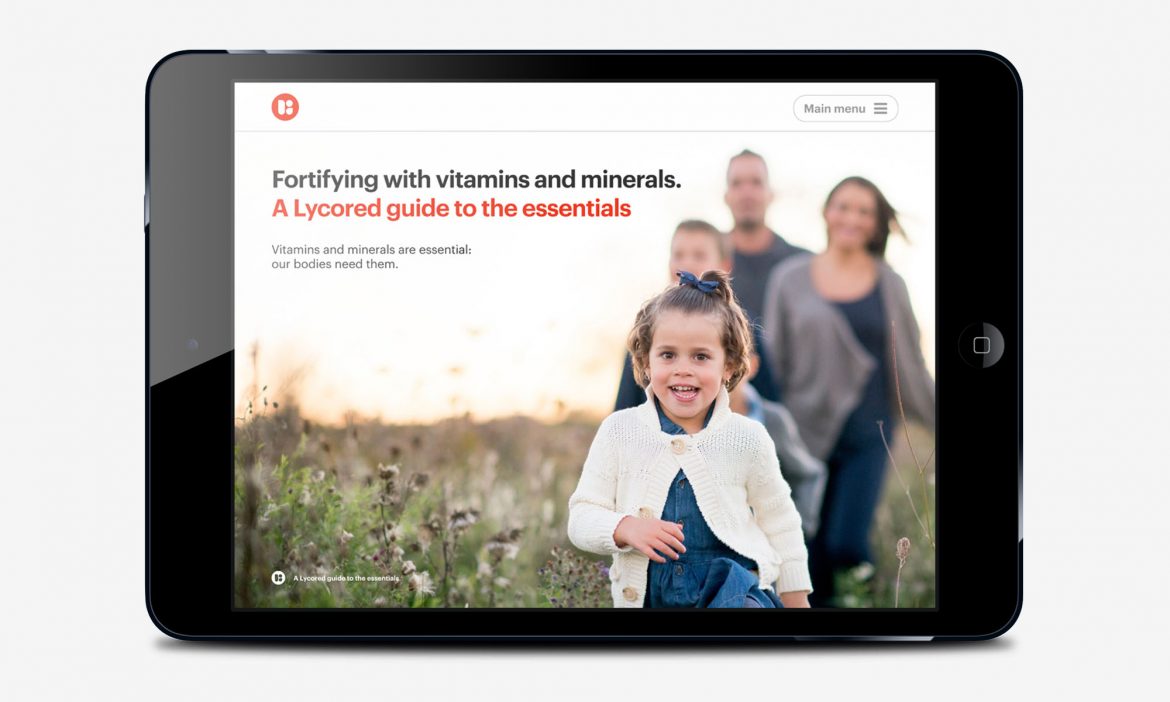Displayed on the black tablet screen is a vibrant image of a family of four in a field bursting with wildflowers. The family consists of a man, a woman, a young boy, and a little girl who stands prominently in the foreground, her beaming smile in sharp focus while her family behind her is slightly blurred. On the right-hand side of the tablet screen, text reads: "Fortifying with Vitamins and Minerals: A Lycord Guide to the Essentials". The text elaborates, "Vitamins and minerals are essential; our bodies need them." Below the image and caption, there is an interface button labeled "Main Menu," distinguishable by three horizontal lines to its left.